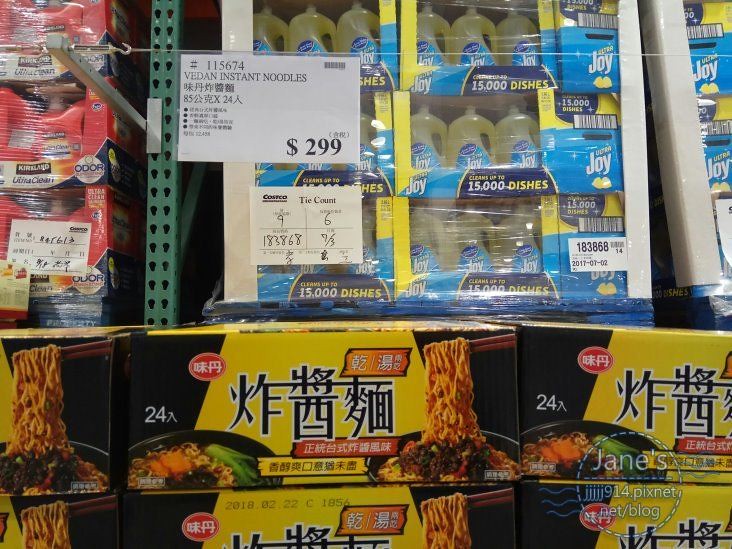In this vibrant image, we observe the bustling environment of a grocery warehouse, reminiscent of Costco, but situated in a foreign country with distinctive Japanese labeling on many products. Dominating the scene is a sign advertising a case of instant noodles priced at $299. The noodle boxes are prominently yellow, featuring mouth-watering images of the noodles themselves. Nearby, a large, unmistakable case of Joy dishwashing soap stands tall; the clear bottles reveal the yellow liquid inside, adorned with blue writing. Additionally, a pink product bearing the recognizable Kirkland brand logo adds a splash of color to the mixture of goods. The diverse array of items, combined with the foreign script, offers a vivid snapshot of an international retail setting.